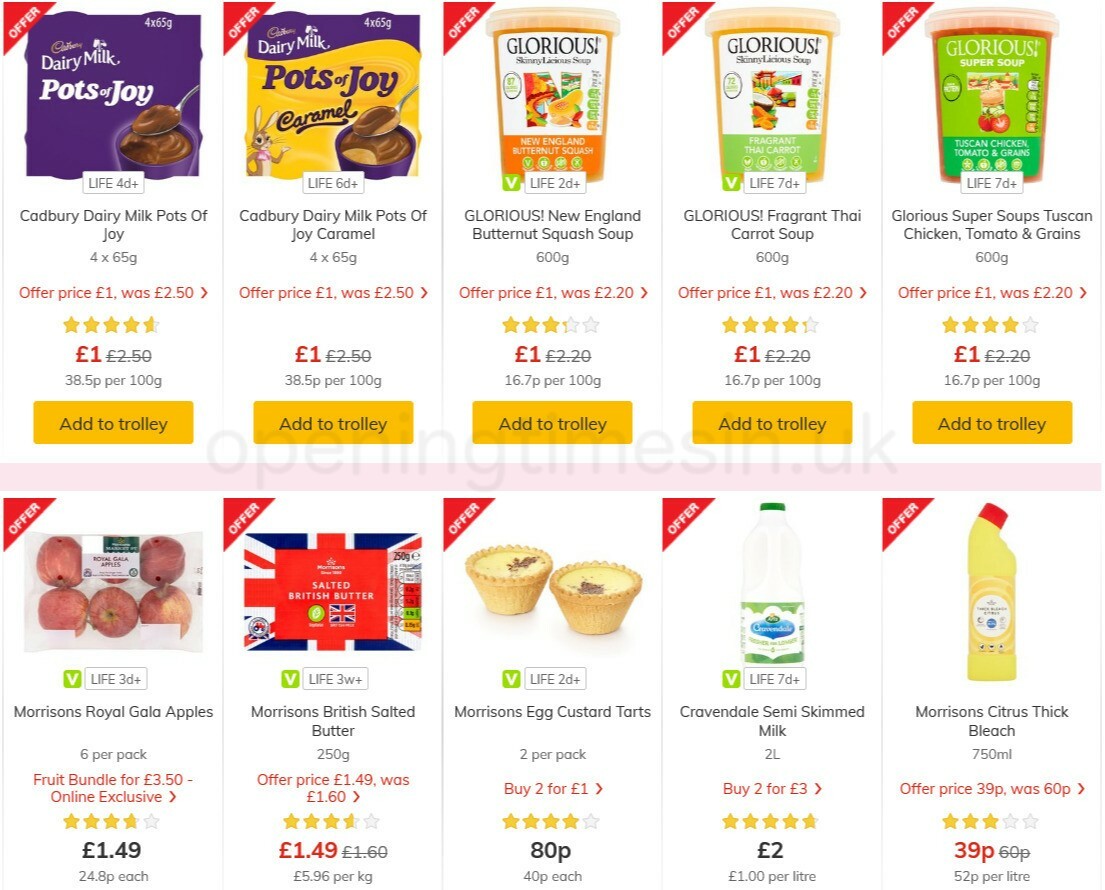The website features a vibrant array of coupons and discounts for a variety of food products, primarily displayed with bright and diverse colors including purple, yellow, green, orange, red, and blue, ensuring a visually engaging experience. A total of ten distinctly colorful food products are showcased, all listed with prices in British pounds, reflecting the European basis of the site.

At the top of the page, a prominently displayed offer features "Pots of Joy" dairy milk desserts, originally priced at £2.50, now available for just £1.00. Following this, another offer for the caramel variant of "Pots of Joy" also appears, similarly discounted to £1.00.

Several types of soups from the Glorious brand are listed:
1. New England Butternut Squash Soup - £1.00
2. Fragrant Thai Carrot Soup - £1.00
3. Super Soups Tuscan Chicken, Tomato, and Grains - £1.00

Other notable discounted products include:
- Morrison's Royal Gala Apples for £1.50
- Morrison's British Salted Butter for £1.50
- Morrison's Egg Custard Tarts for £0.80
- Cravendale Semi-Skimmed Milk for £2.00

These offers provide a broad selection of affordable food items, from fresh produce to dairy and ready-made soups, appealing to a variety of tastes and dietary needs.